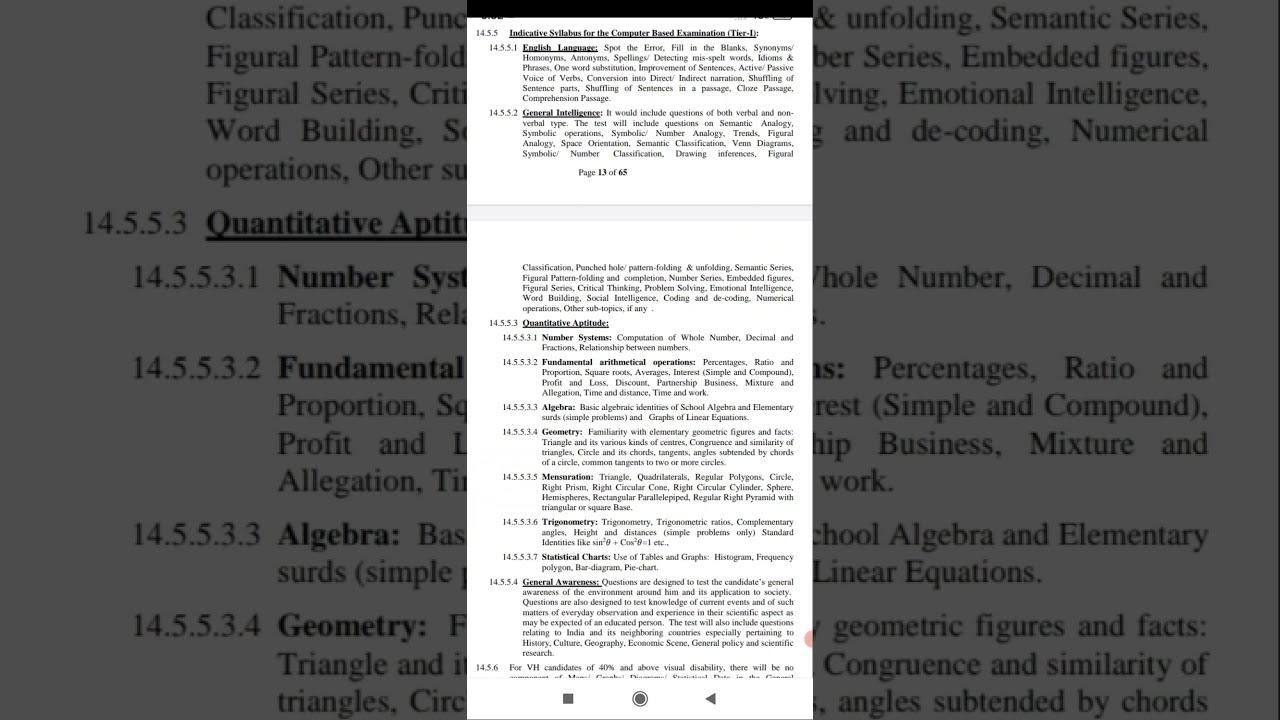This is an image of a book page or a mobile screenshot displaying an outline of the indicative syllabus for a computer-based examination, likely Tier One. The page, seen from a distance and partially cropped, is filled with black and white text, with a mix of small and bold print. The visible text includes numbering systems such as "one four three five" and detailed page numbers like "13 of 63" or "13 of page 65." The main section titled "Quantitative Aptitude" features a variety of mathematical and reasoning topics including number systems, fundamental arithmetic operations, algebra, geometry, decimal figures, fractions, geometric figures, similarity of triangles, elementary business mathematics, mixture and compound problems, simple and compound ratios, numerical operations, percentages, profit and loss, simple and linear equations, and statistical charts. Additionally, the margins are filled with similar terminologies such as figural patterns, embedded figures, classification, unfolding, semantic series, decoding, and emotional intelligence. The layout suggests that the elements in the border are an enlarged image of the central text, enhancing the readability of key terms and section delineations.